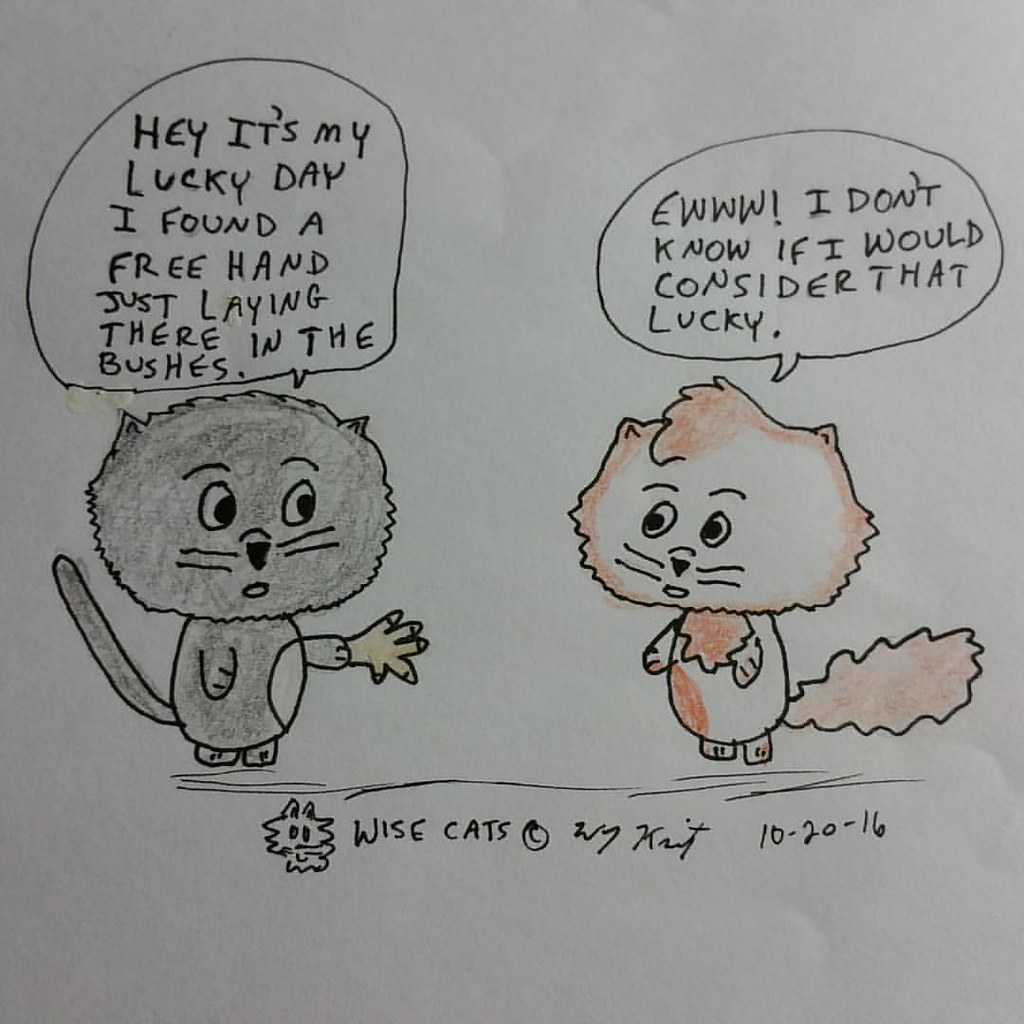This is a square cartoon drawing on a beige background featuring two cats. The first cat, gray in color and on the left, has its hand out and exclaims, "Hey, it's my lucky day! I found a free hand just laying around in the bushes." The second cat, primarily white with pink patches, responds with a look of disgust, saying, "Ew, I don't know if I'd consider that lucky." Speech bubbles containing their dialogue are positioned above their heads. The drawing is detailed with black ink and includes a signature at the bottom reading, "Wise Cats @ Wise Cat 10-20-2016," indicating the artist's handle and the date of creation. The entire image is consistently rendered on a piece of white paper with black lettering.